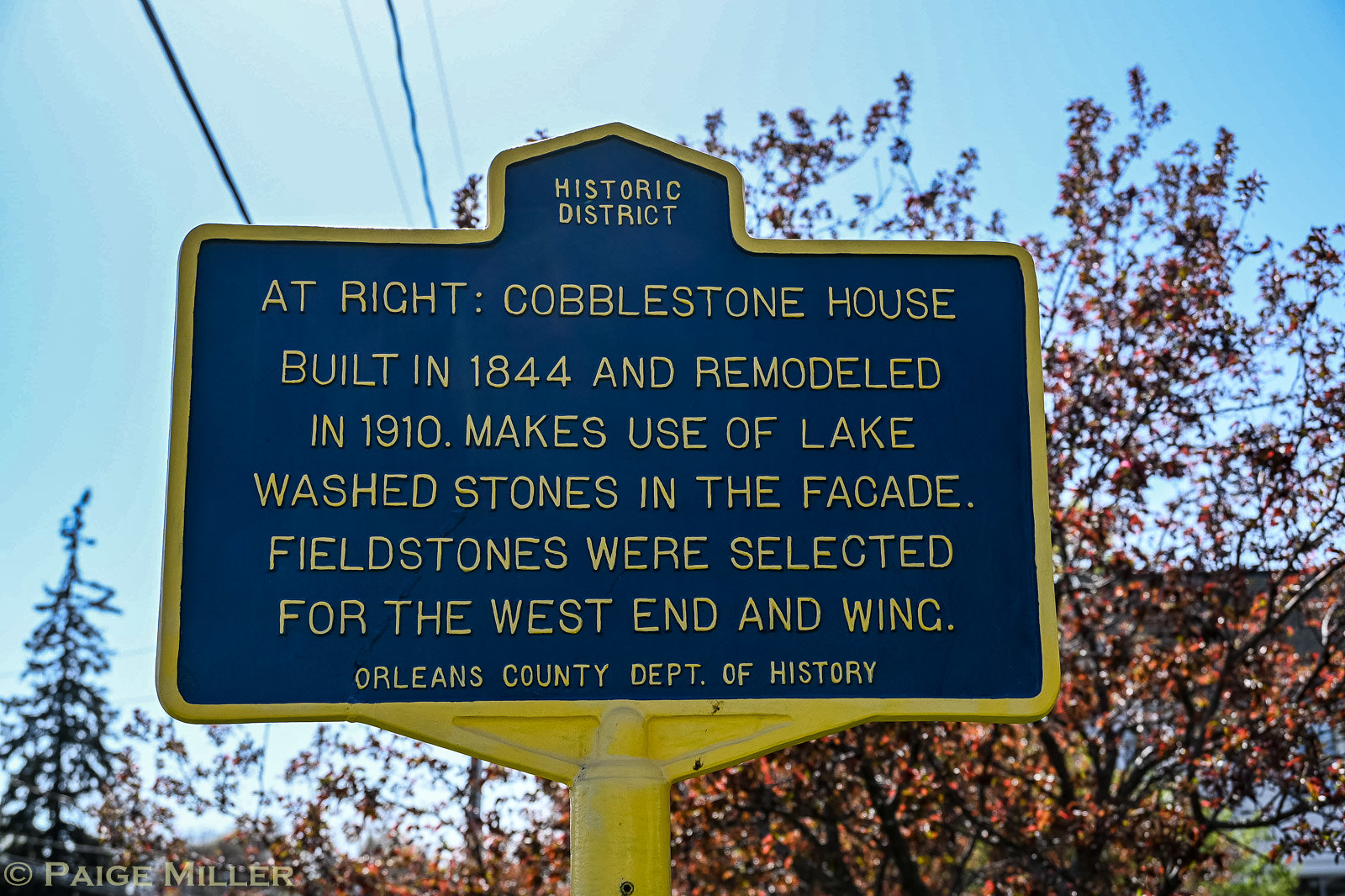This outdoor photograph, taken on a sunny day with clear, blue skies, features a monument plaque prominently displayed on a yellow-trimmed metal stand. The sign, with its bold yellow border and lettering on a dark blue background, stands in front of a bush exhibiting vibrant orange leaves. To the upper left of the frame, power lines are visible running across the image. The plaque reads: “Historic District at Wright Cobblestone House, built in 1844 and remodeled in 1910, makes use of lake-washed stones in the façade. Field stones were selected for the west end and wing. Orleans County Department of History.” Behind the sign, you can catch glimpses of multiple trees and a part of the historic building itself. The sign is firmly planted in the ground, marking a location in a historic district, possibly within a park or town center.